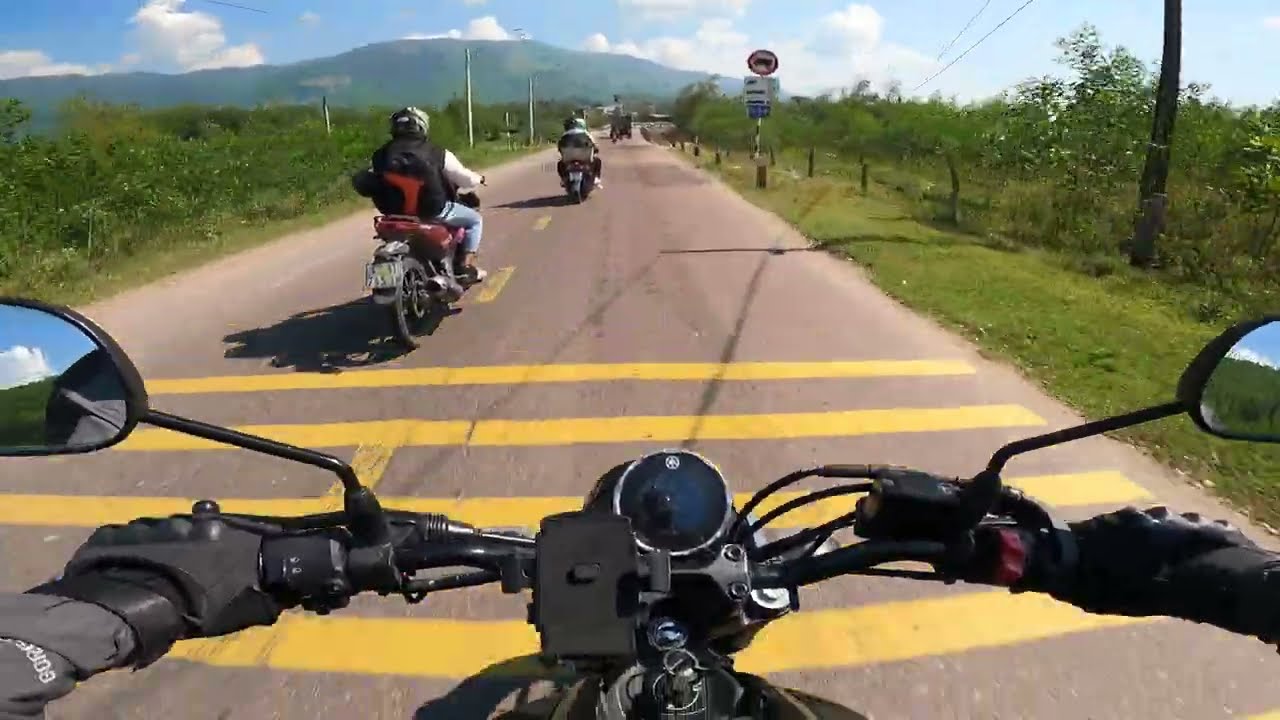The image captures a vibrant, sunlit scene from the perspective of a motorcyclist. The foreground is dominated by the black handlebars of the motorcycle, adorned with dark gloves on both grips. Grey sleeves are visible on the left hand. Attached to the handlebars are two rear-view mirrors, reflecting a picturesque view of greenish-brown mountains, a blue sky, and white clouds. The road beneath is light brown with thick orange and yellow stripes. 

Ahead, another rider on a red motorcycle, clad in blue jeans, a black vest, white sleeves, and a black-and-white helmet, is traveling the same route. Beyond this rider, a third individual on another red motorcycle can be seen, wearing a grey shirt as they blur into the distance. On the right side of the road, there is a yellow road sign on a white pole, and further ahead, another sign with some indistinct markings is visible.

Surrounding the roadway on both sides are stretches of green grass, dotted with small trees and shrubs. In the distance, tall silver poles rise from the ground on the left-hand side. The background showcases majestic, forested mountains topped with clouds, under a largely clear blue sky. It's an expansive scene, rich with natural beauty and the thrill of the open road.